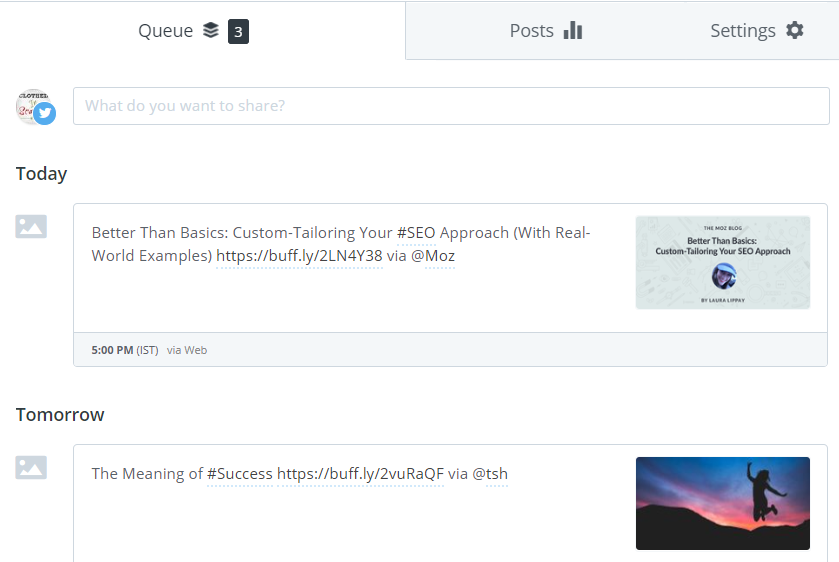The image is a screenshot featuring various elements. At the top of the screenshot is a white background with the word "QUEUE" in bold, black letters. Below the word are three small black diamonds stacked vertically with white space between them. Adjacent to these diamonds is a black square containing the number "3".

To the right, there is a light gray section that includes the words "Posts" and "Settings". Below this, there is a small circular image with some indistinct text and a tiny image inside, which is difficult to discern. Overlaying this circular image is a blue circle featuring a bird, symbolizing Twitter (or now X).

Beneath these elements, there is a long search bar with the placeholder text, "What do you want to share?". Below the search bar, in darker print, is the word "Today". Under this heading is a text box with the title "Better Than Basics: Custom Tailoring Your SEO Approach with Real-World Examples" followed by the URL "https://buff.ly/2LN4Y38" and the attribution "via @Moz".

Further down, under the heading "Tomorrow", another text box includes the title "The Meaning of Success" along with the URL "https://buff.ly/2VURAQF" and the attribution "via @TSH".